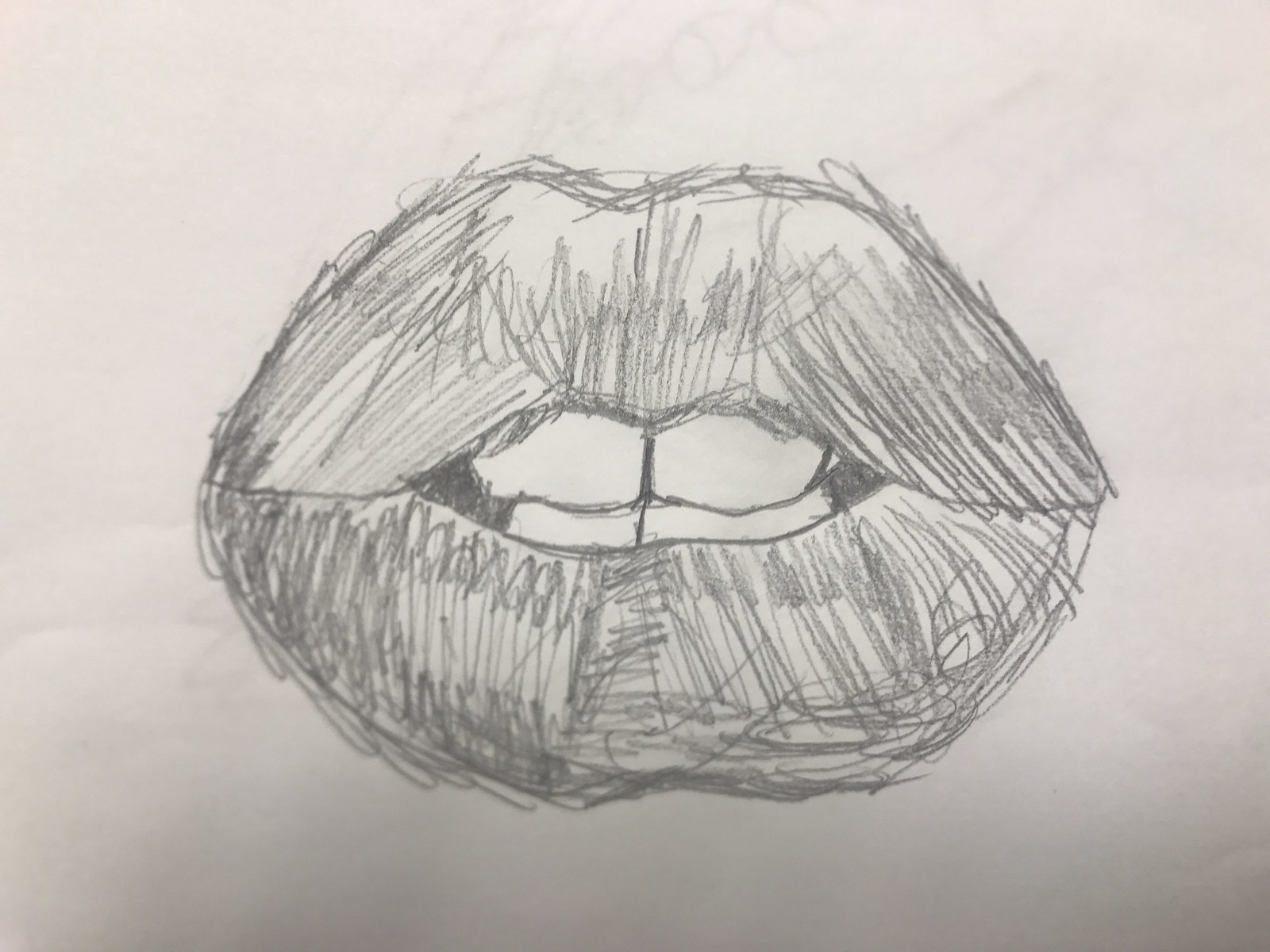This drawing on white construction paper notably features a gradient effect, with the bottom portion of the paper being notably darker than the top. At the center of the composition, a pair of lips has been meticulously illustrated using pencil in shades of black and gray, creating a striking black-and-white effect. The lips are depicted in a somewhat haphazard style, with lines that do not strictly adhere to typical boundaries. Within the lips, four teeth are visible—two on the top and two on the bottom. The corners of the mouth are filled in with solid black, enhancing the contrast and depth of the rendering. The overall image is minimalist, focusing solely on the detailed and expressive depiction of the lips.